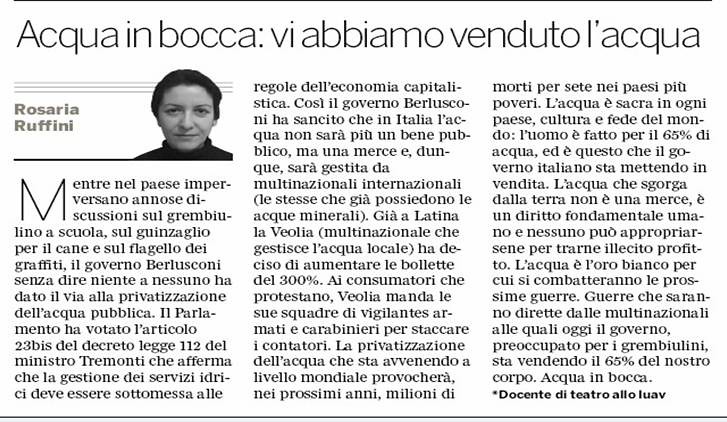The image depicts a newspaper article featuring three columns of neatly arranged black text on a white background. The article is framed by thin horizontal black lines at the top and bottom, providing a clean, defined border. The headline, "Acqua in Bocca vi abbiamo venduto l'acqua," is prominently displayed just below the top border in bold black text. Below the headline, in the upper left corner, is a black-and-white photograph of a middle-aged woman with short black hair, wearing a black turtleneck. Her name, Rosaria Ruffini, is written to the left of the image, which itself is accentuated by three horizontal gray lines behind her head and an additional horizontal black line beneath the photograph. The article appears to be written in a language that resembles either Spanish or Italian, though its exact content is not discernible from the image alone. Concluding the article, in the bottom right corner, an asterisk is followed by the bold phrase "di consente di tetro allo l'uev," which stands out from the rest of the text.